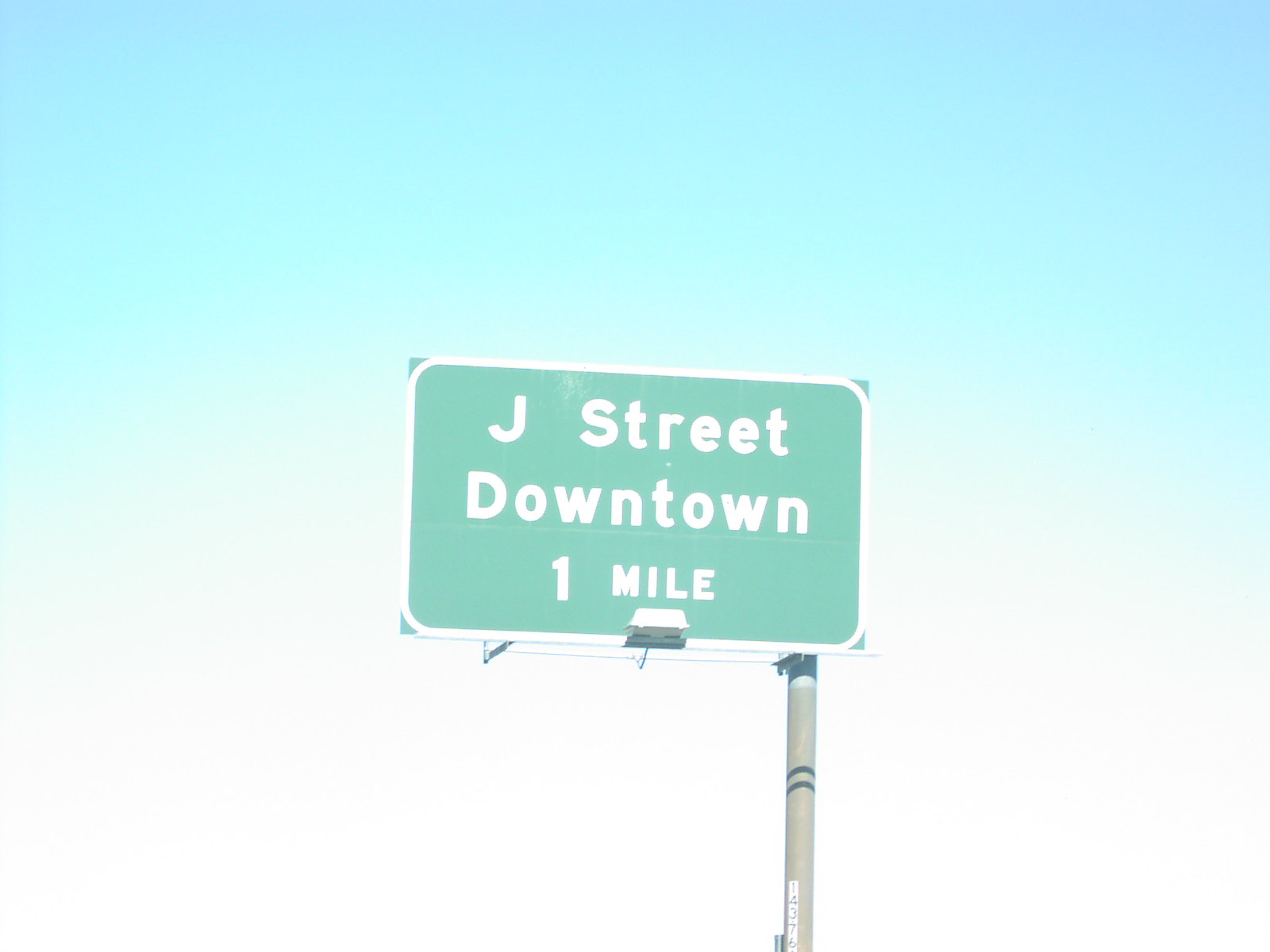This image captures a tall, green rectangular street sign with white trim, mounted on a long gray metal pole situated to the right of the sign. The sign reads "J Street downtown one mile" with the text composed of "J," "Street," "Downtown," and "MILE" being capitalized. The sky in the background features a gradient from a vivid blue at the top to a white, cloud-like appearance at the bottom. The scene includes a small light at the bottom center of the sign, likely intended to illuminate the sign at night. Additionally, there is a double ring band around the pole and a vertical white strip with unreadable text. The minimalist background focuses attention on the sign, creating a striking visual against the sky.